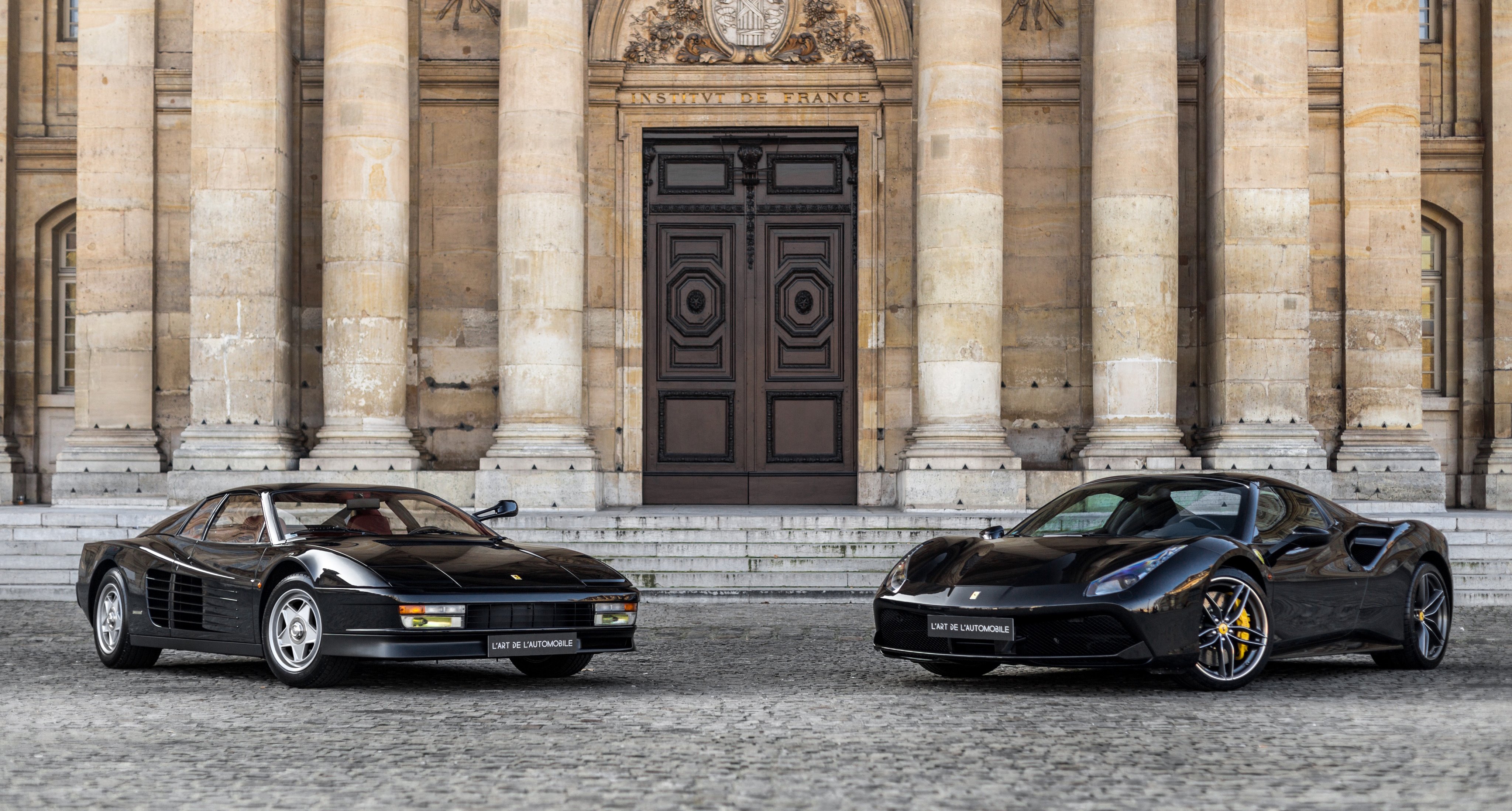In front of the historic Institut de France, which is constructed from slightly weathered, cream-colored stone, two luxurious black sports cars are prominently displayed. The elegant building boasts a grand, arched doorway with the inscription "Institut de France" above its ornate wooden doors. Flanking the entrance are stone columns, and a raised stairway invites visitors inside the majestic structure. The sports cars, likely Ferraris, are artistically positioned at an angle towards each other on a ground of gray cobblestones, each featuring a placard that reads "Le Art d'Automobile," hinting at an appreciation for the artistry of automotive design. The classical, European architectural elements, including the antique columns, suggest a rich historical backdrop, possibly from the classical Greek or Roman revival period.